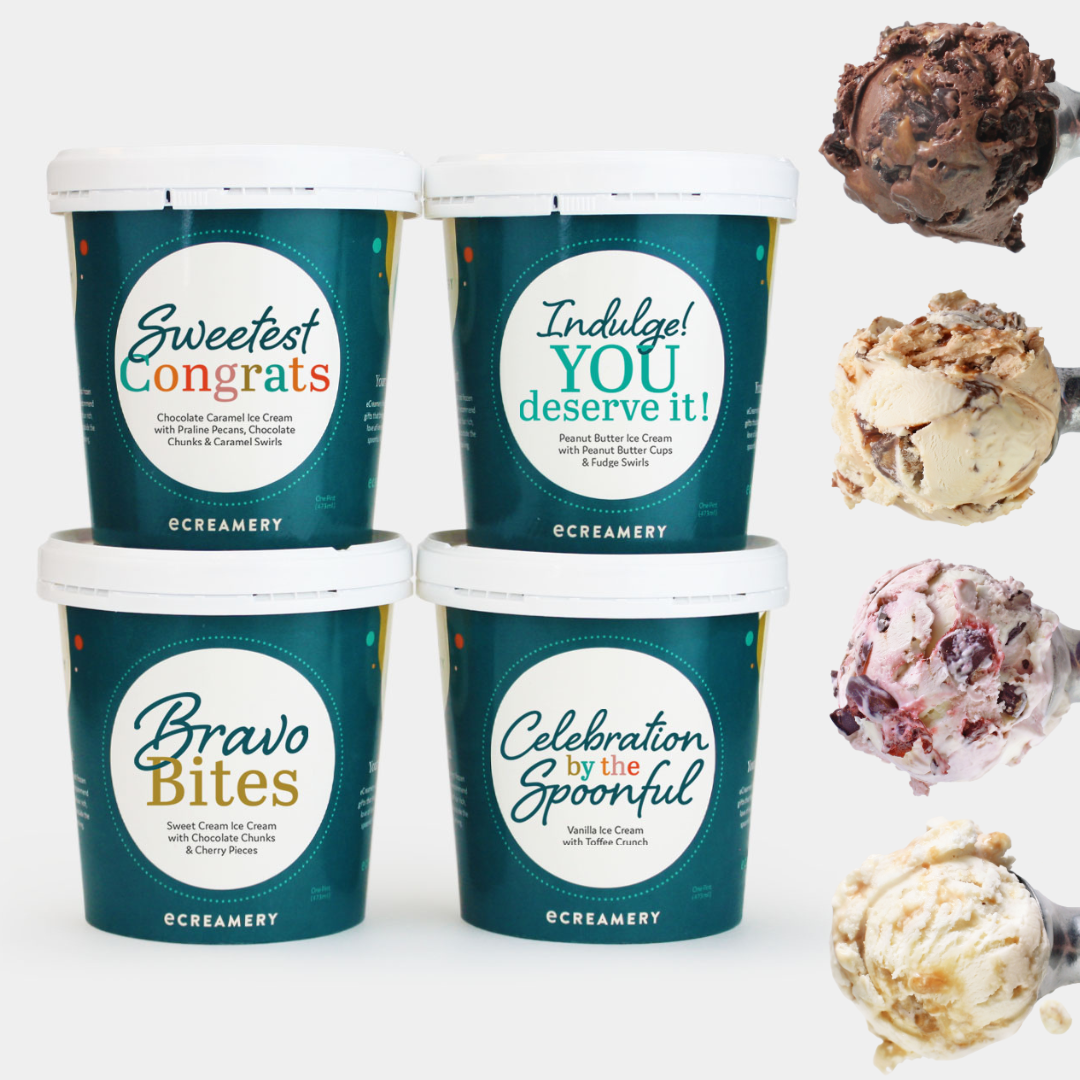In this promotional indoor image, taken under artificial lighting and set against a light gray background, four quart-sized tubs of E Creamery ice cream are neatly stacked two by two. Each container features a distinctive midnight green teal cover with a white lid and a central white circle displaying the name of the ice cream. The top left tub is labeled "Sweetest Congrats: Chocolate Caramel Ice Cream with Praline Pecans, Chocolate Chunks, and Caramel Swirls." Below it is "Bravo Bites: Sweet Cream Ice Cream with Chocolate Chunks and Cherry Pieces." In the upper right, the tub is labeled "Indulge, You Deserve It: Peanut Butter Ice Cream with Peanut Butter Cups and Fudge Swirls." The lower right tub reads "Celebration by the Spoonful: Vanilla Ice Cream with Toffee Crunch."

On the far right of the image are four metal scoops, each holding a single serving of one of the ice cream flavors. From top to bottom, the scoops respectively display a chocolatey mix with crunchy pieces, a butter almond-like flavor, a strawberry mix with nuts, and another probable variation of butter almond. The brand, E Creamery, is consistently emphasized, showcasing the delectable and diverse selection of ice cream flavors such as chocolate, butterscotch, strawberry, chocolate chip, and vanilla.